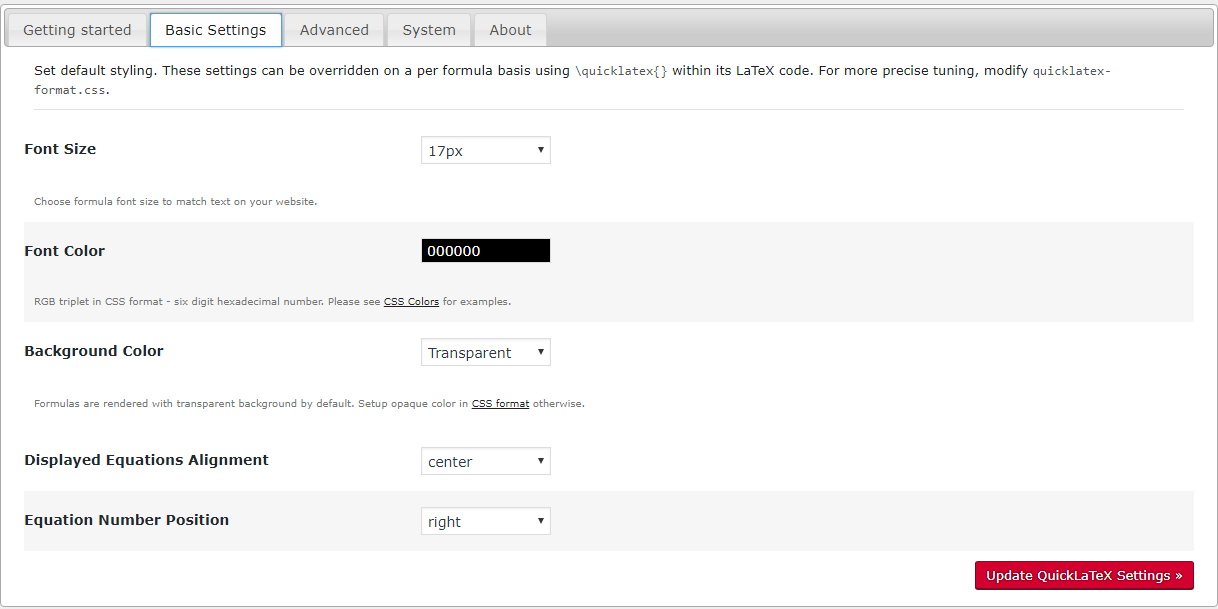The screenshot captures a section of a website with a predominantly white background, accented with some gray elements. At the top of the screenshot, there are several navigation tabs labeled "Getting Started," "Basic Settings," "Advanced System," and "About."

The "Basic Settings" tab is active, revealing a detailed interface for configuring default styling options. Below the tab header, there's an instructional note stating, "Set default styling. These settings can be overridden on a per formula basis using QuickLaTeX within its LaTeX code. For more precise tuning, modify quicklatex.format.css."

The settings presented include various adjustable parameters:
1. **Font Size:** Set to 17 px, with a note that advises users to "choose formula font size to match text on your website."
2. **Font Color:** Set to black (represented by all zeros, #000000).
3. **Background Color:** Set to "transparent," ensuring the formula blends seamlessly with any website background.
4. **Displayed Equations Alignment:** Currently set to "center," allowing users to adjust the alignment of equations within the text.
5. **Equation Number Position:** Configured to appear on the "right" side of the equation.

Each setting is accompanied by menus or options that users can utilize to make further adjustments, ensuring their displayed mathematical formulas integrate smoothly and appear consistently across their website.